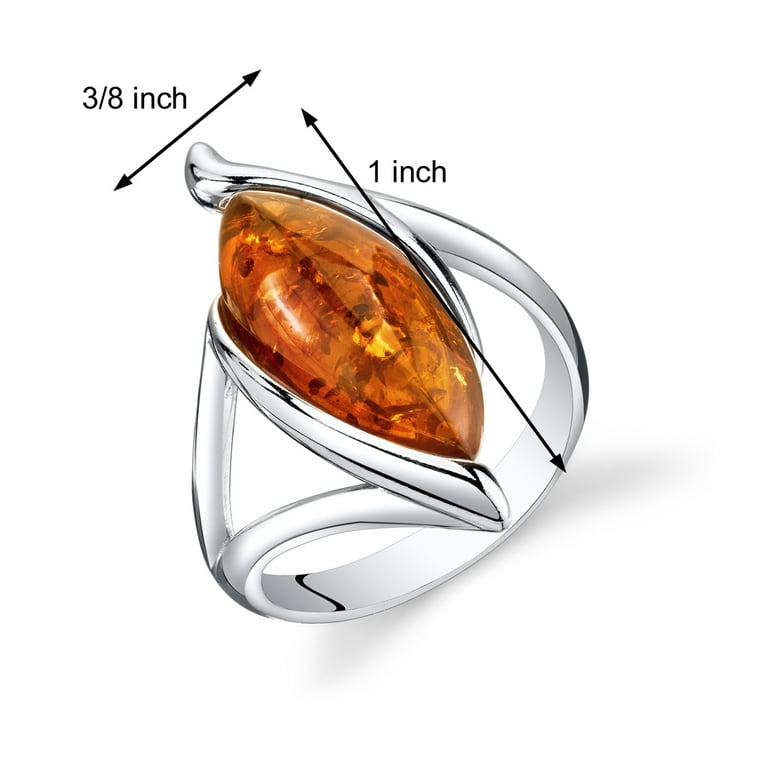This image showcases a uniquely designed silver ring featuring an oblong, football-shaped gem at its center. The gem varies in description, appearing amber with goldish-orange hues and striking dimensions, although some may perceive it as brown and unappealing. The ring's band is solid at the back, with an artistic structure that rises over the gem on one side and dips down to create a triangular opening on the other. Precise measurements accompany the design, with black arrows indicating a width of one inch from bottom to top and three-eighths inch across the top. The entire visual is set against a solid white background.